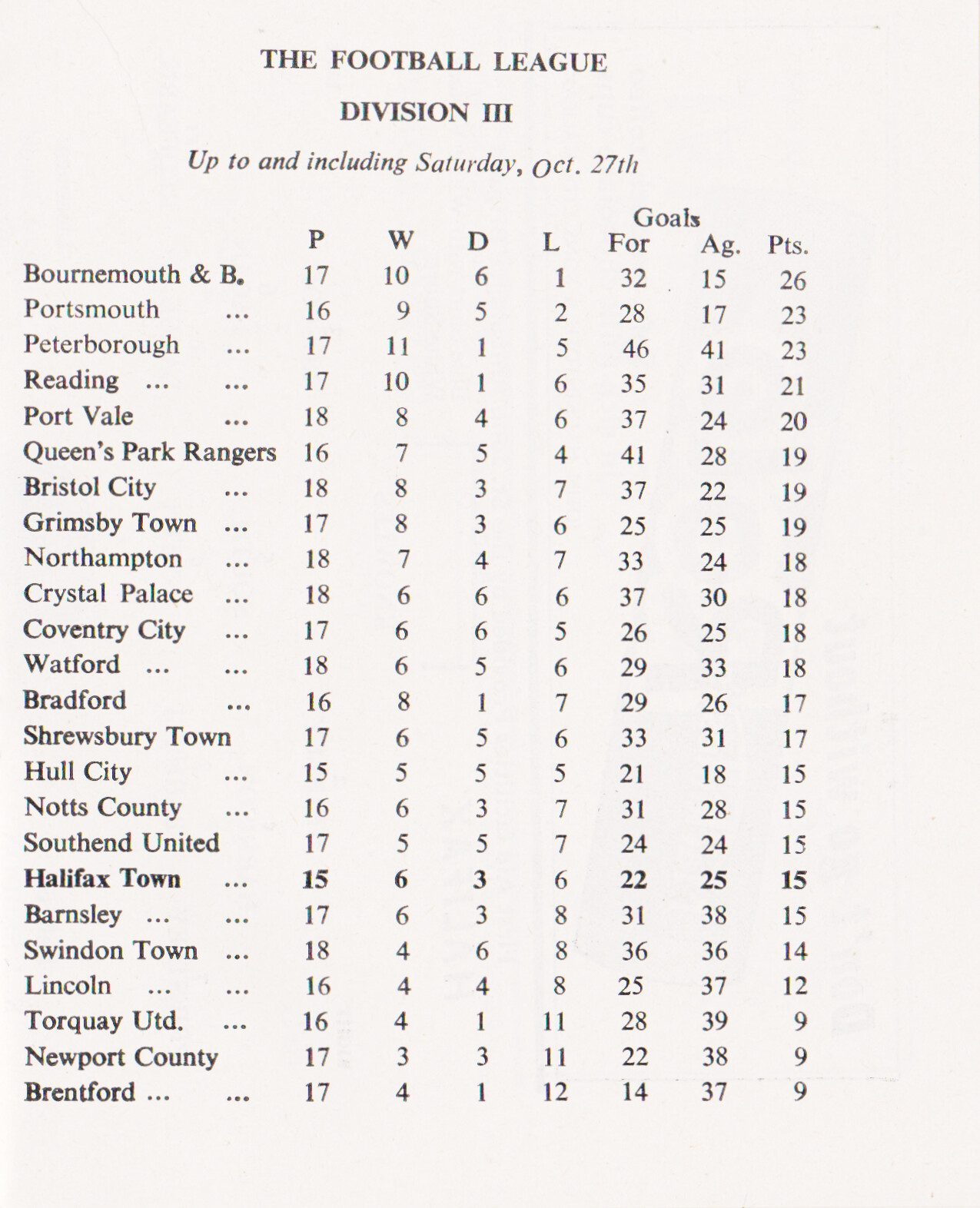The image is a detailed print of the Football League Division 3 standings up to and including Saturday, October 27th. The data is presented in black text on plain white paper, using a Times New Roman font. The standings list team names along the left-hand margin, including teams like Bournemouth and Boscombe Athletic (referred to as Beauremont, 8 and B), Portsmouth, Peterborough, Reading, Port Vale, Queens Park Rangers, Bristol City, Grimsby Town, Northampton, Crystal Palace, Coventry City, among others. Each team's performance is detailed across several columns marking 'P' (possibly played games), 'W' (wins), 'D' (draws), and 'L' (losses), along with goals scored 'For' (GF) and 'Against' (GA), and their total points.

The sheet meticulously outlines that Bournemouth and Boscombe Athletic lead with 26 points, followed by Portsmouth and Peterborough, both tied with 23 points. Reading has garnered 21 points, and Port Vale holds 20 points. In stark contrast, at the bottom of the standings, teams like Torquay United, Newport County, and Brentford are tied with just 9 points each.

This stat sheet is comprehensive in recording each team's games played, wins, draws, losses, goals scored (both for and against), and total points, providing a clear picture of the league's standings as of October 27th.